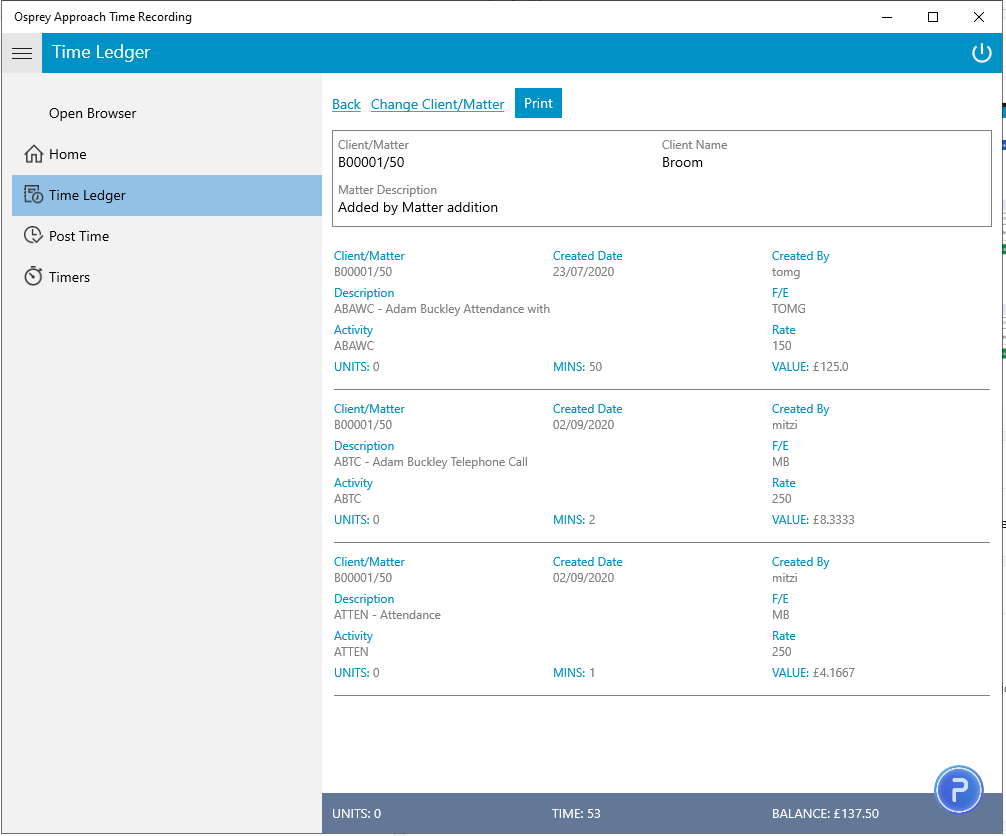**Detailed Caption:**

The screenshot displays the Osprey Approach Time Recording interface. At the very top, there is a small text header beneath which a blue line of code runs horizontally. On the left side of the screen, within a gray box, there is a hamburger menu icon followed by the label "Time Ledger" highlighted in blue, indicating an active selection. 

To the left of the interface, there is a vertical menu system with the following options: "Open Browser," "Home," "Time Ledger" (highlighted in blue), "Post Time," and "Timers." 

To the right of the menu, there are functional buttons labeled "Back," "Change Client Matter," and "Print." Below these buttons, within a highlighted rectangular area, detailed information about a client matter is displayed:

- **Client Matter**: B0001-50
- **Matter Description**: Added by Matter Addiction
- **Client Name**: Broom

Subsequent entries are listed in similar highlighted areas, detailing various activities:

1. **Description**: ABAWC (Activity by Adam Buckley)
   - **Activity**: Adam Buckley Attendance With
   - **Creator**: Tom
   - **Creation Date**: [Unknown]

2. **Description**: Adam Buckley Telephone call
   - **Creator**: Mitzi
   - **Creation Date**: [Unknown]

3. **Description**: Attendance
   - **Creator**: Mitzi
   - **Creation Date**: [Unknown]

At the bottom of the interface on a lavender background, summary details are noted:
- **Units**: 0
- **Time Recorded**: 53
- **Balance**: 137.5 British Pounds

The interface appears to be a part of a time tracking and client management system, capturing detailed logs and descriptions of various client-related activities.